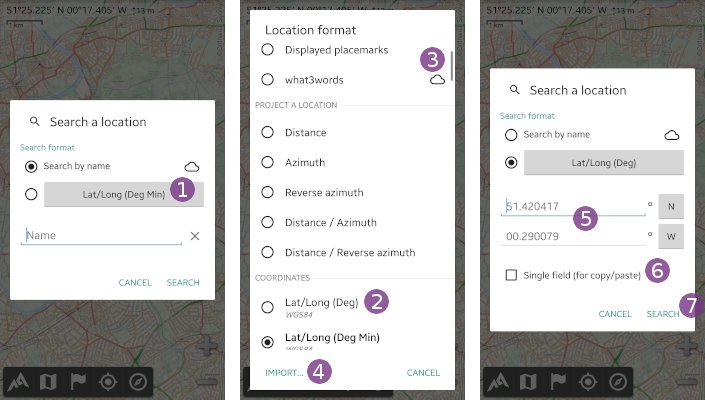A composite image of three screenshots from a GPS app on a mobile device, showing different interfaces within the app:

- **Left Screenshot**: The interface displays the "Search for a location" feature. The user interface includes a "Search Format" section, where "Search by Name" is selected by default. Below, there's an option to search using "Lat/Long DEG-MIN," accompanied by a filled-out field. A prominent purple button sits adjacent to this field. There is an empty "Name" field below this, flanked by "Cancel" and "Search" buttons. The background features a partially visible map.

- **Center Screenshot**: The "Location Format" interface is displayed, offering various location input options. There are two sub-sections: "Project a location" with several coordinate input options, and another section. Labels "2," "3," and "4" in purple indicate specific elements: "2" highlights the coordinates option "Lat/Long DEG," "3" is near the "What3Words" option denoted by a cloud symbol, and "4" marks an "Import" button.

- **Right Screenshot**: The user returns to the "Search for a location" interface, but this time the "Lat/Long DEG" option is selected for the search format. Coordinate fields for latitude and longitude have been populated. Purple labels "5," "6," and "7" are marked diagonally across the interface, indicating key interactive points: "5" at the top left, "6" further down at the bottom right, and "7" at the bottom right corner.

Overall, the images illustrate the app's different ways to input and search locations, emphasizing ease of use with visibly marked interactive elements.